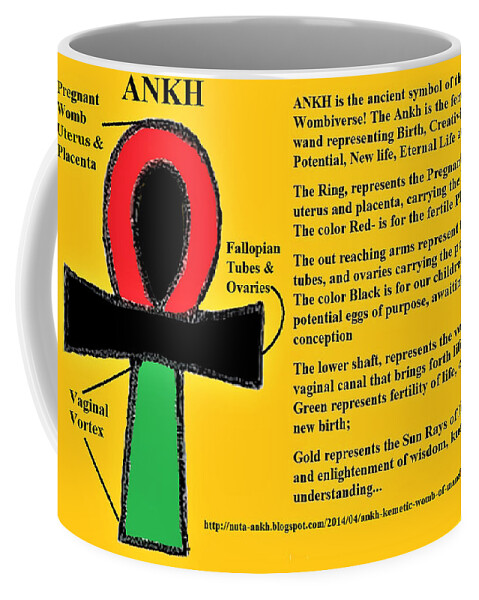This detailed photograph showcases a ceramic coffee mug with a vibrant yellow exterior and a white interior, accompanied by a contrasting white handle partially visible on the left side. Dominating the mug's bright yellow body is a meticulously illustrated ankh symbol. This symbol, resembling a cross with a round, curved top, is artistically segmented into three distinct, color-coded sections: the top, colored red and labeled "Pregnant Womb, Uterus, Placenta"; the middle, colored black and inscribed with "Fallopian Tubes and Ovaries"; and the bottom, colored green and marked "Vaginal Vortex." Surrounding the ankh, there is extensive black textual content, explaining, "The Ark [Ankh] is the Ancient Symbol of the Wombiverse. The Ark is the Wand representing Birth," followed by key terms like "Potential, New Life, and Eternal Life." Additional smaller text and a website URL are located towards the bottom but are mostly illegible in the image.